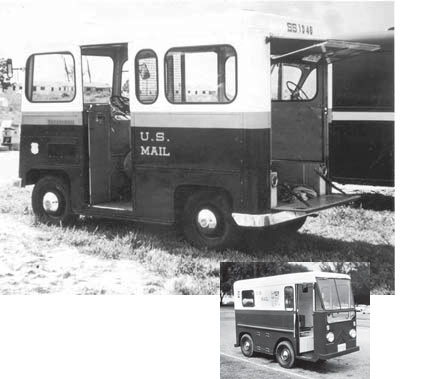The image is a pair of vintage black and white photographs of the same U.S. Mail van, presented side-by-side within a small white border. The larger photograph at the top captures the van from a side-rear perspective, revealing its dual-tone design with a darker bottom and a lighter top. The van's back is open, showcasing its tailgate and upward-folding windshield, suggesting a hatchback functionality. Multiple rectangular windows are visible along the van's sides. Parked on a grassy field, the backdrop includes a glimpse of nature and possibly other vehicles.

The smaller, lower photograph provides an alternate view of the same van, focusing on the driver's side where the sliding door is noticeable. Unlike the top image, the doors and windows in this view are closed, offering a clearer look at the van's front headlights and detailed features like the license plate and windshield wipers. Both photographs, steeped in a grayscale palette, convey a nostalgic, historical essence, seemingly from the early to mid-1900s. The intricate depictions include the US Mail insignia and subtle differences in window arrangements, reinforcing the vehicle's bygone era and utilitarian purpose.